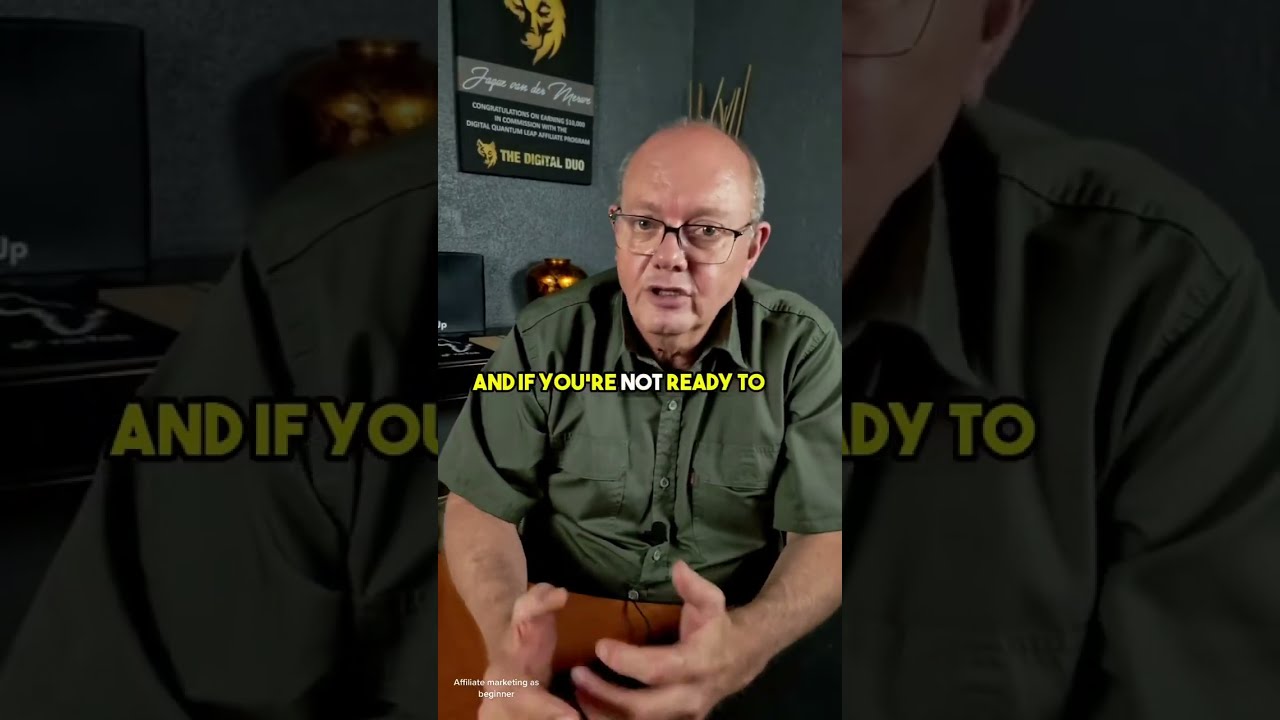In the image, the central focus is an older Caucasian man with balding, white hair closely cropped on the sides, wearing thin black metal glasses and a button-up, short-sleeve shirt in shades of green or khaki. He is positioned at the center of the picture, seemingly speaking directly to the camera. His hands are extended forward in an open, grasping motion. A line of text overlays his chest, fragmented as "and if you're" in yellow, "not" in white, and "ready to" in yellow. In the background, part of an office setting is visible with a gray wall and a poster on the left side, partially readable with the words "The Digital Duo." The image format suggests it may be a screenshot from a social media app like TikTok, featuring a mirrored effect where the left and right thirds display enlarged sections of the central image, showing partial repetitions of the man's shoulders, face, and the text.